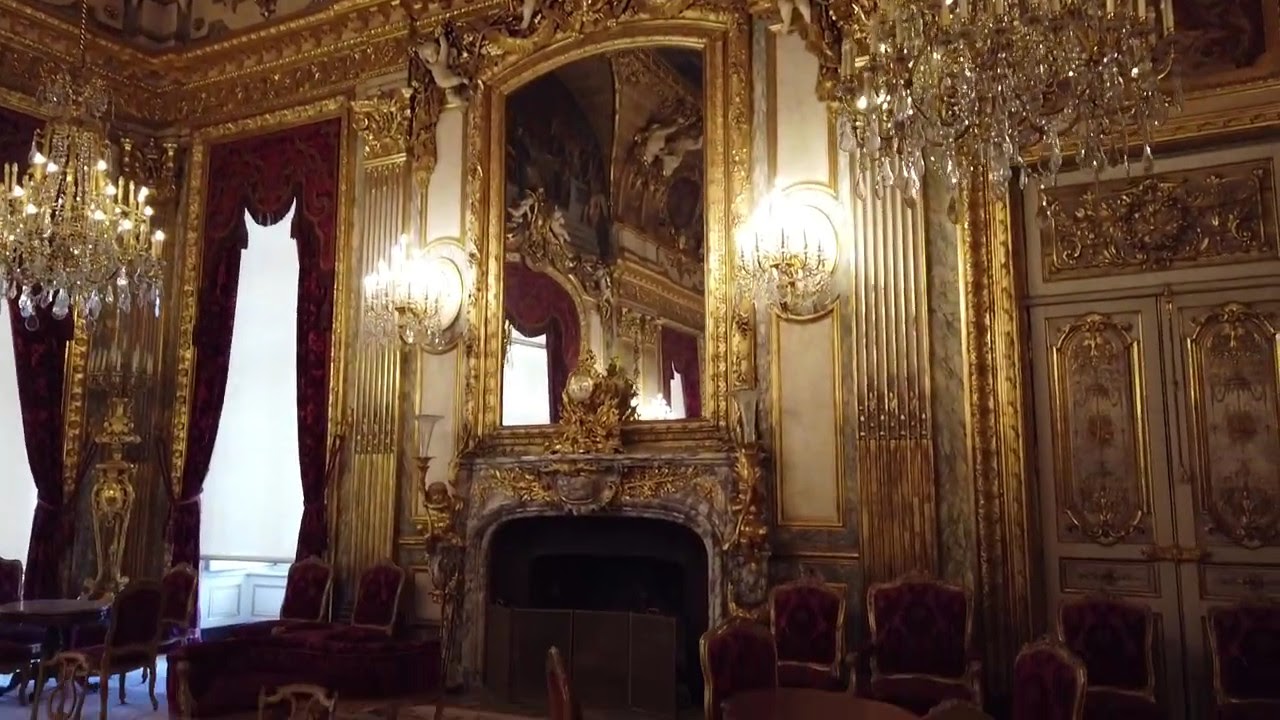This detailed landscape-orientation photograph captures the opulent interior of a grand palace or castle. The focal point is a large ornate wall adorned with intricate golden designs, with a grand arched gilded mirror positioned above a carved mantle fireplace. Crystal sconces flank the mirror, casting a brilliant glow. Crystal chandeliers hang majestically from the ceiling, one on the far left and another to the upper right. Rich red velvet drapery frames the windows, through which natural light streams despite the shades being partially drawn. The lavish room features brown tables and red-cushioned chairs, highlighting the scale and grandeur of the space where the fireplace toweringly dwarfs the chairs. The lavish decor, gilded door frames, and sumptuous details vividly exemplify the room’s luxurious aesthetic.